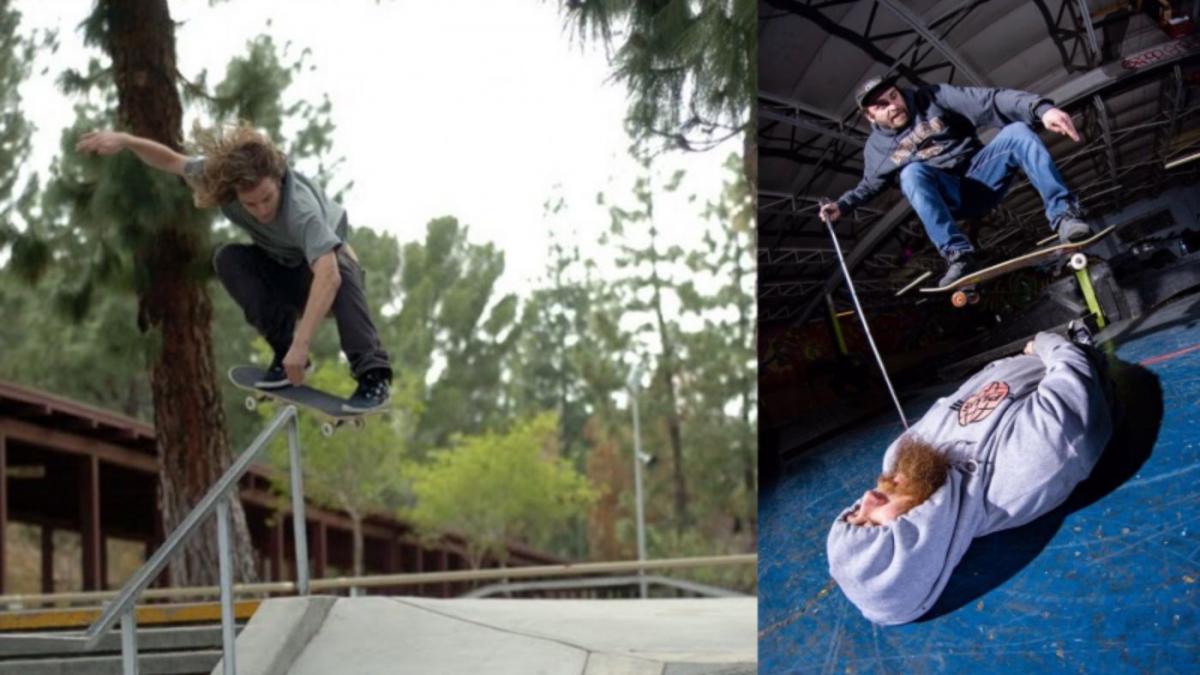These are two photographs positioned side by side, capturing dynamic skateboarding scenes. The left photograph depicts a white man with long curly red hair, donning a gray short-sleeved shirt and black pants, executing a board slide down a metal rail adjacent to cement stairs. This outdoor scene is framed by a lush backdrop of scotch pine trees and a partial wooden awning to the left. His knees are bent, his right arm is extended outwards for balance, and his left arm is directed forward. The right photograph takes place indoors, possibly in a warehouse skate park with a blue linoleum floor. It captures a dramatic moment as a skateboarder, dressed in blue jeans, a gray hoodie, and a hat, jumps over another man lying face-up on the floor. The prone man, who has a scruffy red beard, is bundled in a gray hoodie with the hood tied tightly around his face, while the airborne skateboarder, with bent knees, navigates the stunt above him. The indoor setting is characterized by a warehouse roof visible in the background.